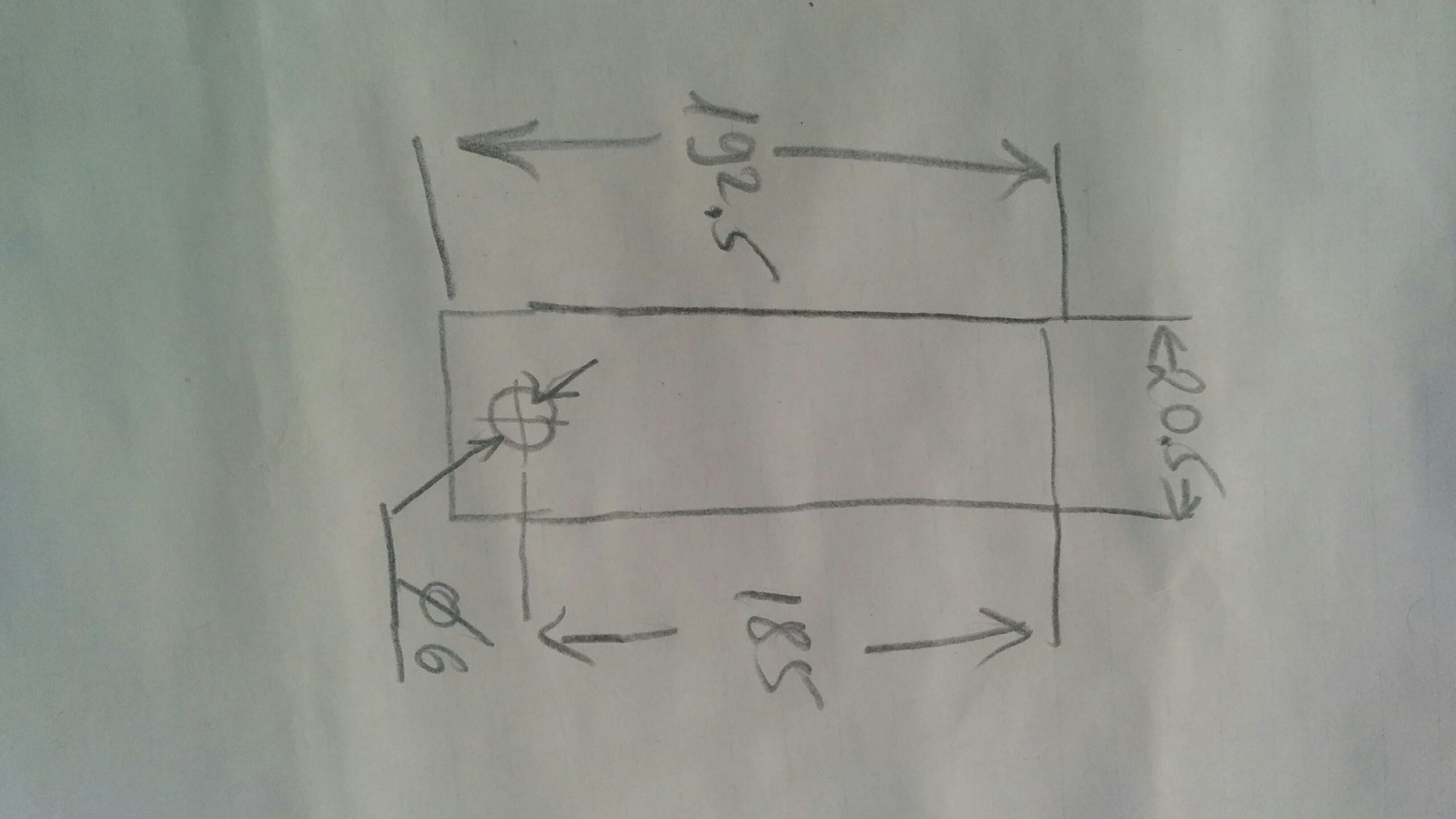The image depicts a detailed pencil line drawing on a blank white sheet of paper, likely representing the location of a particular object with multiple precise measurements marked. 

At the center of the drawing is a rectangle with several lines and arrows illustrating various dimensions and directions. 

- On the north end of the rectangle, there are two vertical lines extending upward beyond the rectangle towards the sky. 
- To the right (east side), a line extends horizontally outward, and slightly above this, another line extends to the left (west), making the left side's lines higher than those on the right. 
- On the left side (west side), another set of lines is drawn horizontally at the end, matching the height where the rectangle ends. The line on the left extends outwards, with its outer line being shorter than the corresponding one on the right.
- Also on the left, there is a double-ended arrow indicating vertical distances, with arrows pointing both south and upwards. Between these arrows, the measurement "192.5" is noted.
- On the right side, an upward arrow extends north with the accompanying measurement "185," and a southward-pointing arrow below indicates a distance marked "0 6" (with the zero crossed by a diagonal line).
- Below the south end of the rectangle, an arrow extends diagonally downwards to a small circle about a centimeter in diameter located at the rectangle's southern extremity. Opposite to this diagonal line, there is another similar arrow pointing towards the same circle.

Returning to the top (north end), where the vertical lines extend upwards, another set of double-ended arrows is present, horizontally pointing east and west. The space between these arrows is marked "20.5," suggesting another measurement. 

Overall, the drawing meticulously maps out spatial relationships and measurements with numerous arrows and annotations, providing precise information about the described object's location and dimensions.